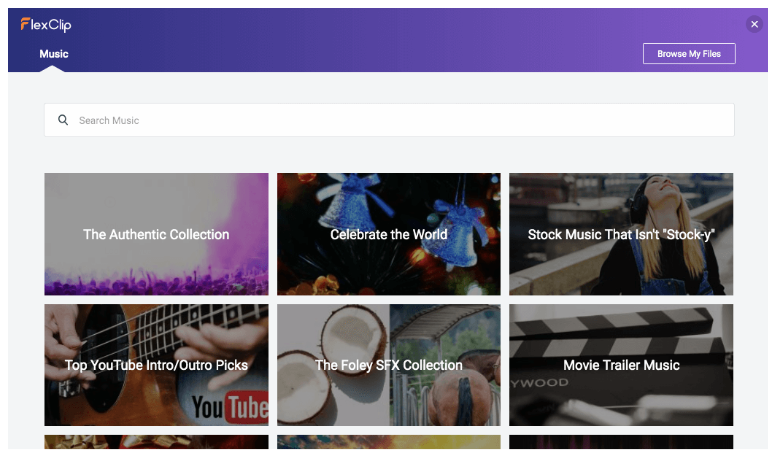**Detailed Caption:**
The image is a screenshot captured from the "FlexClip" website, displayed in landscape mode as seen on a monitor or laptop screen. The topmost portion of the image features a blue navigation bar, which transitions from a dark navy blue on the left side to a lighter cobalt blue on the right. On the left side of this bar, the website's logo is prominently displayed. The logo reads "FlexClip," with a red 'F' and white letters for the rest of the word, and the 'C' in "Clip" is capitalized. Adjacent to this logo on the top right corner is a white circle containing an 'X,' indicating a close button for the screen.

Beneath the blue navigation bar, the background shifts to a very pale blue hue. The search functionality is represented by a long, white search bar stretching almost across the entire width of the screen. Inside this search bar, to the left, there is a magnifying glass icon followed by the placeholder text "Search Music."

Below the search bar, there's a curated selection of music categories, each represented within a rectangular card displaying photographs with overlaid white labels. The first row contains:
1. **"The Authentic Collection"** - The image features a crowd of concert-goers, evoking a lively music concert atmosphere.
2. **"Celebrate the World"** - The photo for this category is ambiguous and hard to discern from the description.
3. **"Stock Music that Isn’t Stocky"** - Depicts a woman with blonde hair, wearing headphones, her head tilted back as she enjoys music. She appears to be seated in a relaxed setting.

The second row includes:
1. **"Top YouTube Intro/Outro Picks"** - Shows a close-up of hands skillfully playing a guitar. The bottom right corner features the YouTube logo.
2. **"The Foley SFX Collection"** - Consists of two photographs: the left image displays a halved coconut showing the white flesh inside, and the right image is unclear.
3. **"Movie Trailer Music"** - Features an image of a classic clapperboard, commonly used in film production, with a backdrop resembling a street sign design.

A further row of categories is visible below but is cropped off in the screenshot, leaving the details of these items obscured.